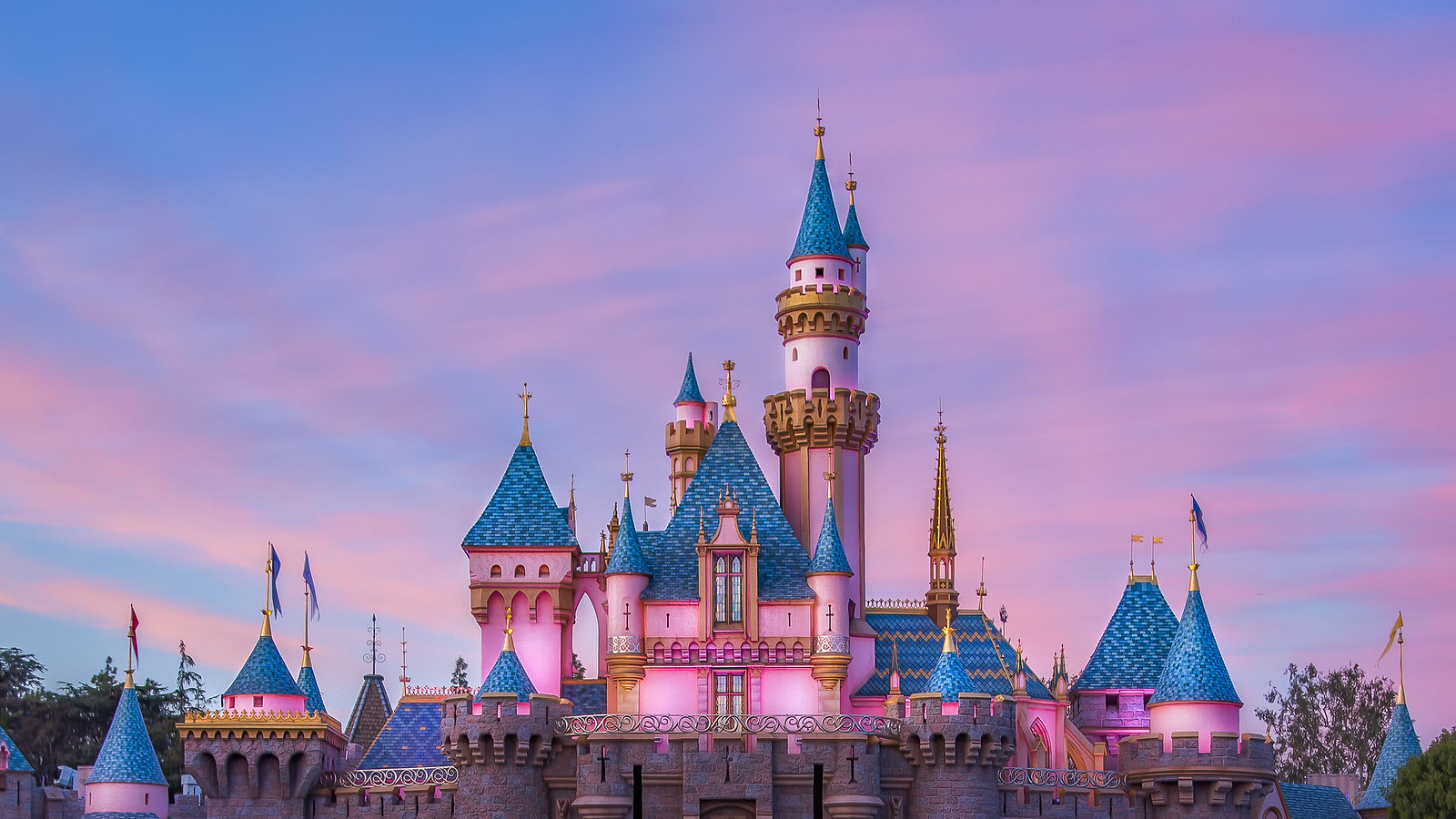This image appears to be a digitally rendered interpretation of Disneyland's iconic castle, possibly inspired by Snow White's castle. The scene showcases the upper portion of the castle under a vibrant blue sky accentuated with pinkish clouds. The castle itself boasts a harmonious blend of bright pink walls and dark aqua blue peaked tile roofs. Roughly eight or nine turrets are adorned with distinct gold crosses, small flags, or gold balls on their steeples, enhancing the castle’s intricate architectural details. Though the entire structure isn’t fully visible, the base suggests a surrounding gate constructed from dark reddish-purple bricks. The scene features some green trees adding to the cheerful and lively ambiance, capturing the essence of a magical, animated utopia.